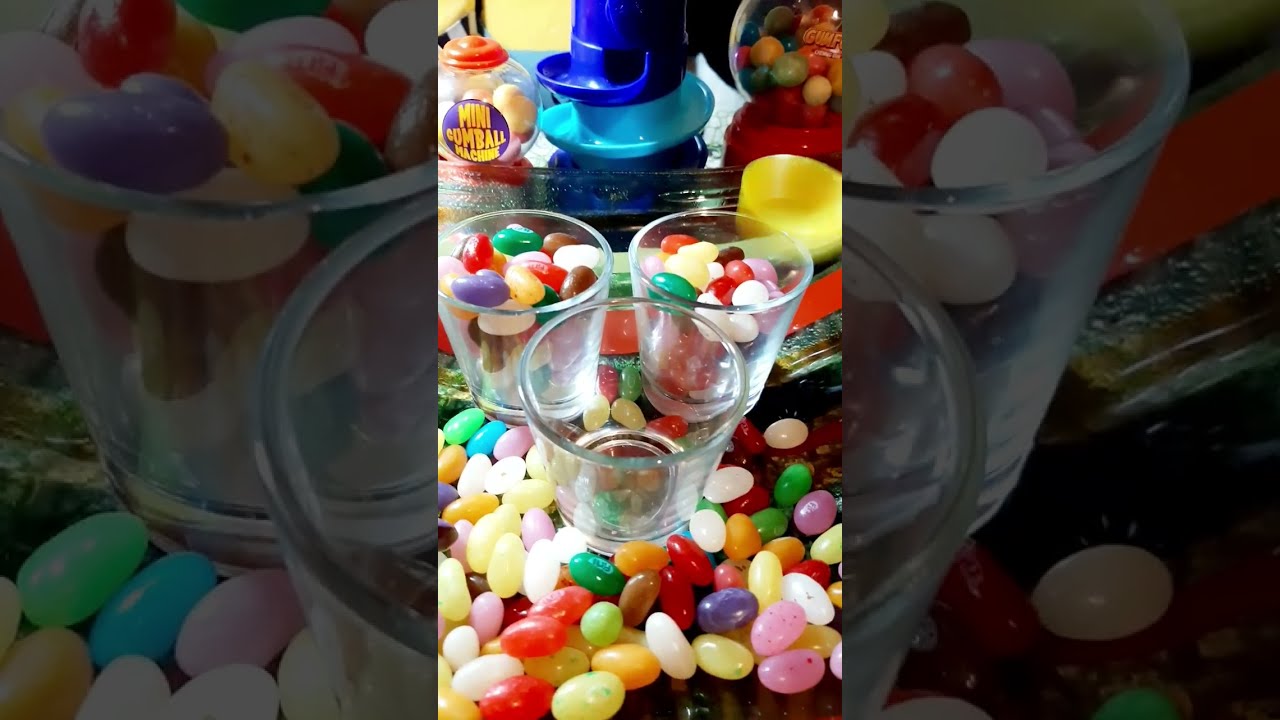In the vertical, vibrant image, three cylindrical shot glasses sit on a shallow pile of colorful jelly beans atop a table. The shot glasses are arranged in a triangular formation: the front one is empty, while the two behind it are brimming with jelly beans. The jelly beans are a delightful mix of red, orange, yellow, green, purple, pink, white, and brown, with some featuring specks. Surrounding the shot glasses, the scattered jelly beans create a lively, vivid scene. In the background, a mini blue gumball machine and two additional gumball machines add depth and a nostalgic charm to the setup, enhancing the image's overall appeal. The bright and varied colors of the jelly beans and the playful arrangement make for an eye-catching display.